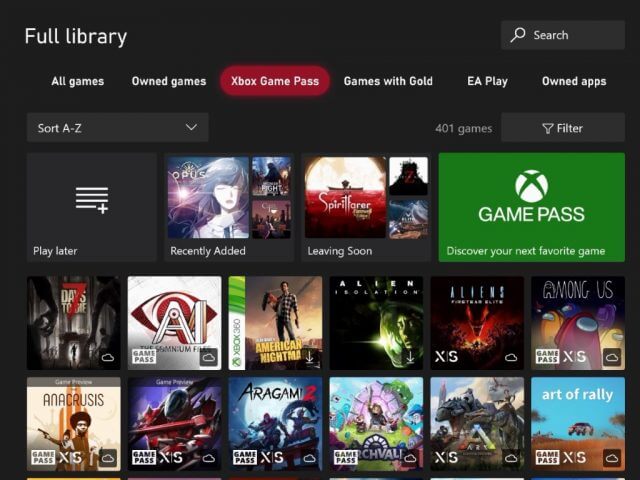The image features a black background with various categories and menus related to Xbox gaming displayed prominently. At the top, it reads "Full Library" followed by options such as "All Games," "Owned Games," "Xbox Game Pass," "Games With Gold," "EA Play," "Owned Apps," "Search," and "Filter." The total number of games is listed as 401, and the sorting option is set to "A to Z" with other filters like "Play Later," "Recently Added," and "Leaving Soon."

Highlighted sections include promotional banners for "Game Pass" with the tagline "Discover Your Next Favorite Game" and a peculiar creature with hands alongside an AI design with an eyeball. The display shows various game categories including "Cloud," "Xbox 360," and specific titles like "American Nightmare" and "Nightmaw," which is ready for download.

One notable visual element includes an alien and a woman in a green astronaut suit, along with the conspicuous "XS" designation for certain games. Further details include a "Red Tornado," characters from "Among Us," and multi-colored thumbs with blue nails. Another feature highlights the game "Anna Cruz's" with visuals of a man with an afro and another holding a pistol against an orange-colored background.

Additionally, a "Game Pass XS" section showcases a robot wielding a sledgehammer, a scene titled "Eragon 2" with characters set against a moonlit backdrop, "Chivalry" featuring a small figure with a sword beside a rock, and "Art of Rally" where a car is seen mid-jump in the air.